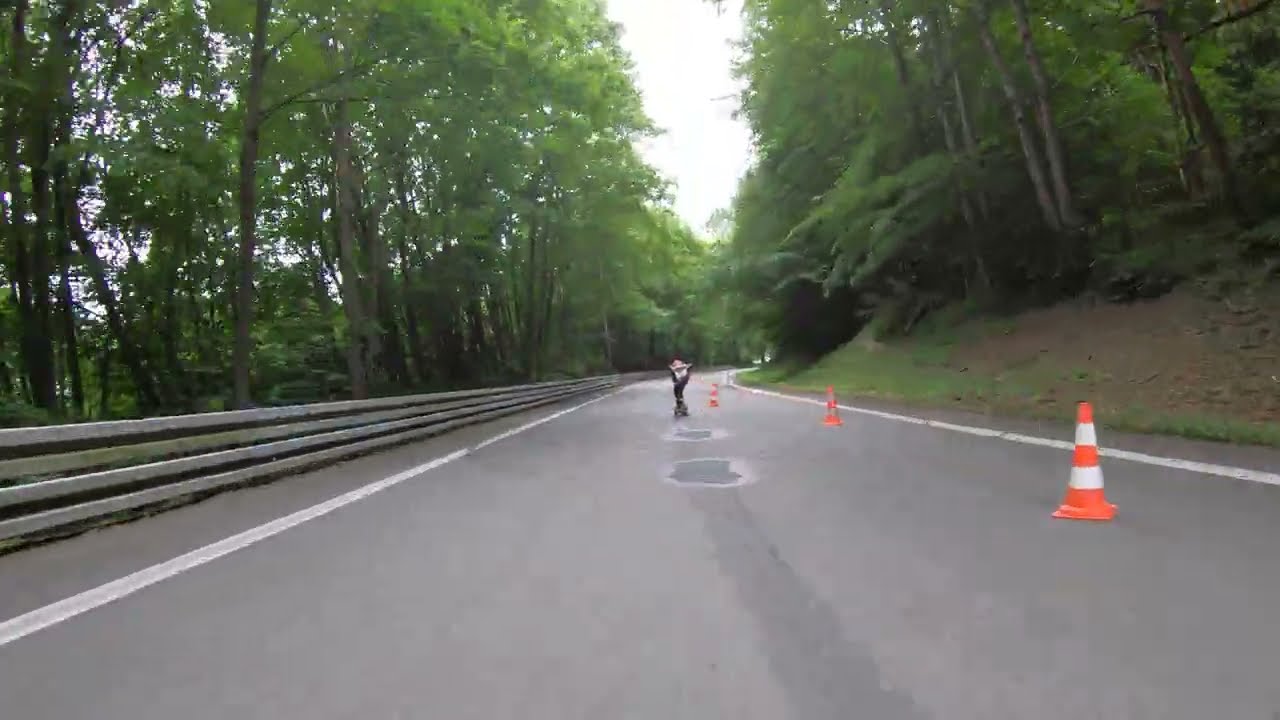The photograph, captured on a bright day after recent rain, depicts a scenic outdoor setting centered on a two-lane road. The road, dark gray and seemingly eroded in the middle where the stripe typically lies, is flanked by vibrant, tall trees on both sides, with some branches forming a natural canopy further in the background. On the right side of the road, the ground rises into a hill, and there are several traffic cones, suggestive of a race or a safety measure. Puddles from the recent rain dot the lane. The left side features a guardrail extending around a curve, preventing vehicles from veering into the thick forest. In the very center of the image, a small, indistinct figure, possibly a person on rollerblades or a skateboard, dressed in black, travels along the road. Sunbeams pierce through the tree branches, illuminating the serene pathway.